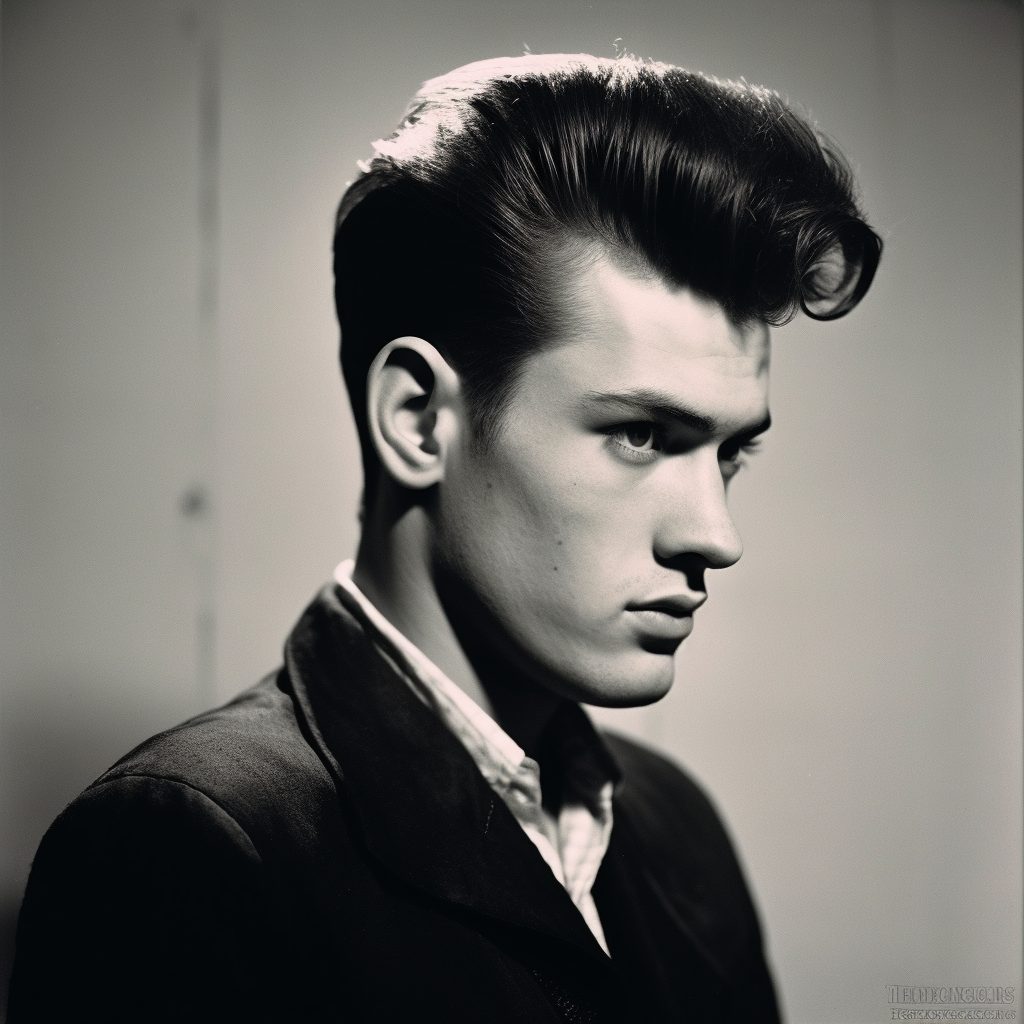This vintage black and white portrait, likely from the 1950s, features a young, handsome man with a serious expression, gazing intently to his left. His dark brunette hair, styled in a classic pompadour with a shiny, perhaps gelled or greased, finish, curls into a loop over his forehead. He sports a white dress shirt beneath a tailored black jacket, suggestive of a formal suit ensemble. The photograph captures a side profile, highlighting his strong facial features and intense stare. The background is a slightly out-of-focus gray, emphasizing the sharp contrast and clarity of his visage. The image, which has the qualities of a professional headshot, includes an indecipherable tag in the bottom right corner, adding to its timeless, vintage appeal.